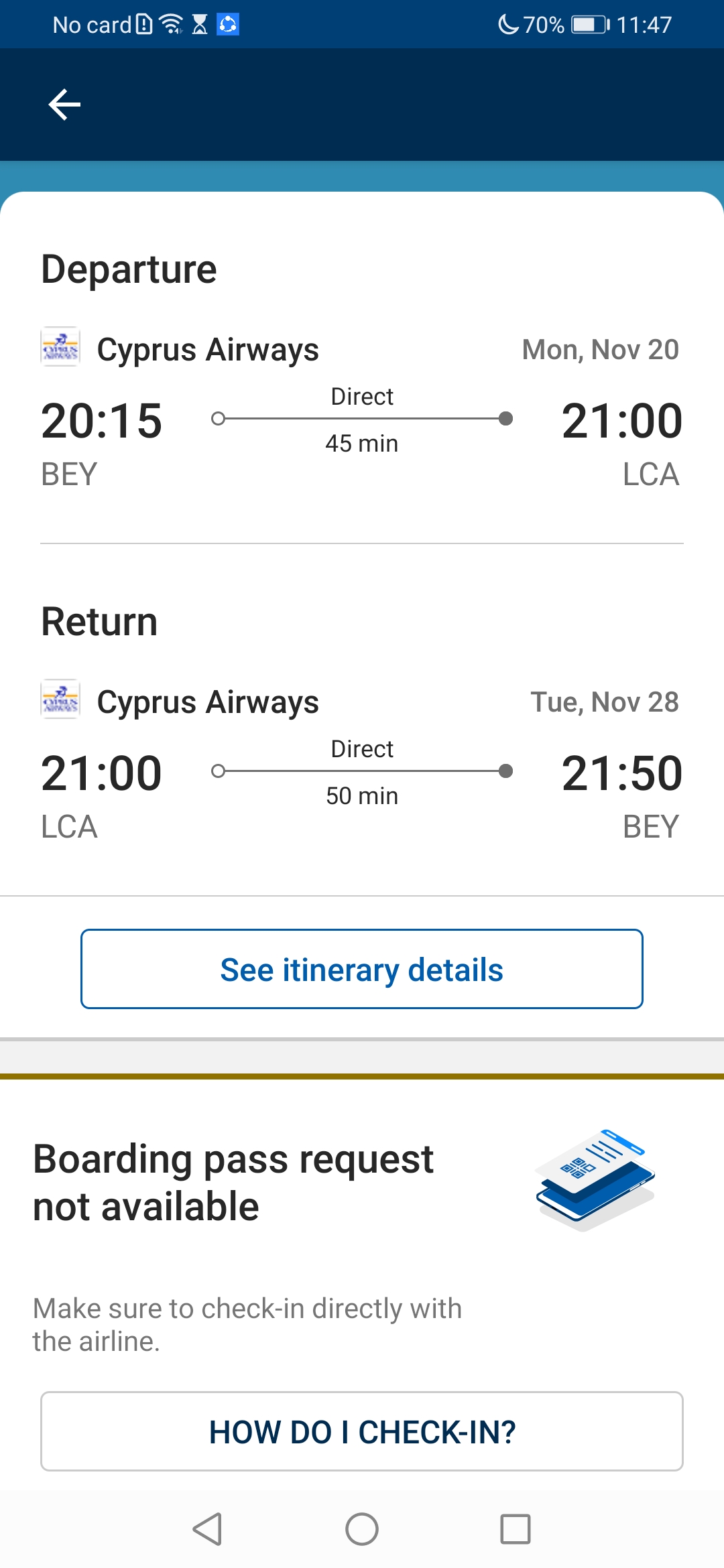This screen capture from a flight booking website details an individual's flight ticket on Cypress Airways. The top section features a dark blue bar, which includes a "No Card" notification, a Wi-Fi signal icon, battery percentage at 70%, and the time displayed as 11:47. Below this, in the white section, the departure information is shown: the airline is Cypress Airways with the flight number 2015 BEY, a direct flight of 45 minutes. The departure date and time are listed on the right as Monday, November 20, at 21:00 LCA. 

Further down, the return flight details are provided: again with Cypress Airways, departing at 21:00 LCA and a direct flight lasting 50 minutes. The return date and time are specified on the right as Tuesday, November 28, at 21:50 BEY. Following this information, there is a button labeled "See Itinerary Details." Underneath, a message indicates that a boarding pass request is not available, followed by another button labeled "How Do I Check In."